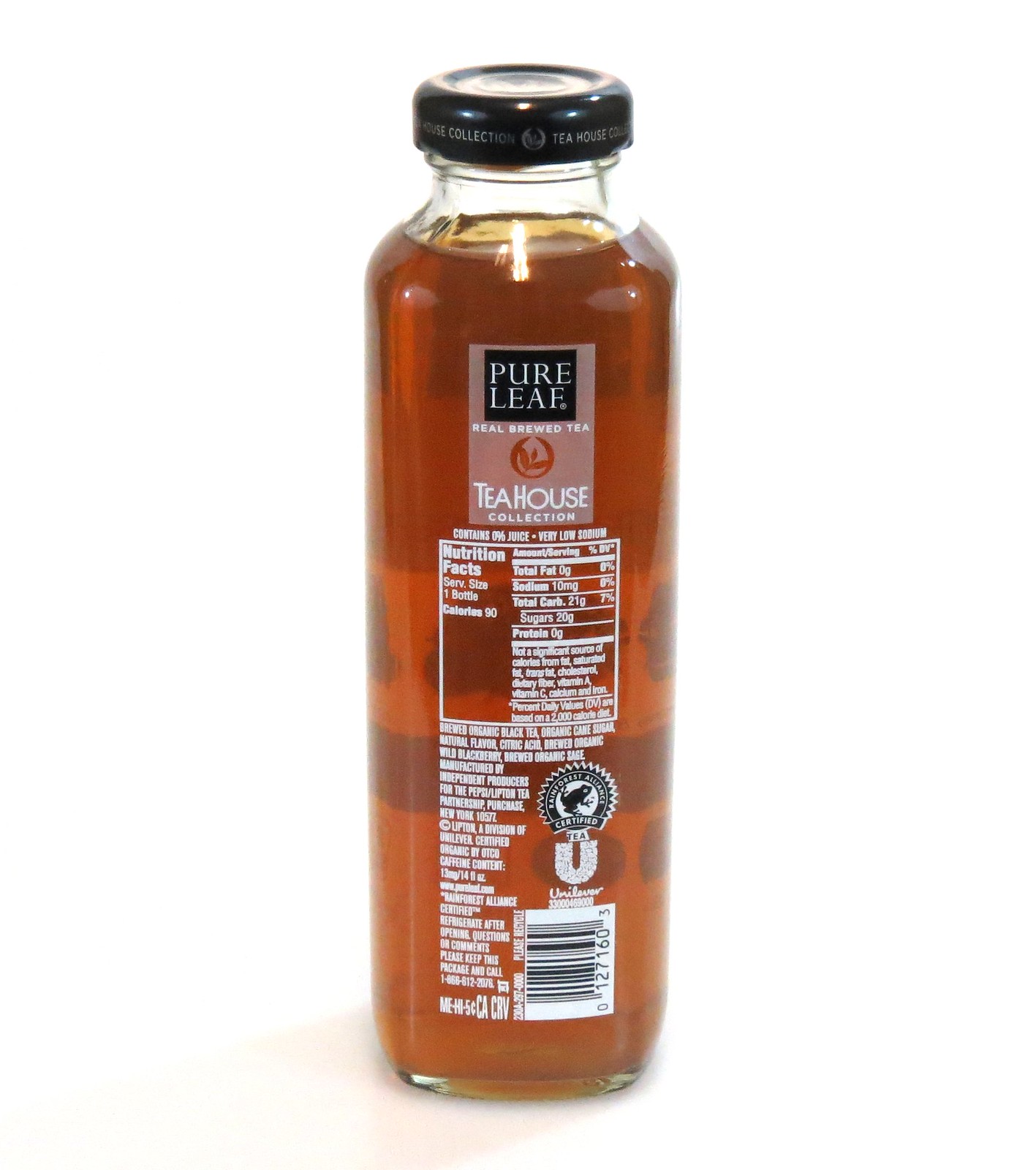This image features a Pure Leaf Real Brewed Tea bottle. The bottle is made of glass and stands approximately six inches tall. We are viewing the back, where the detailed product information and nutrition facts are displayed. The bottle tapers at the top to a black screw cap, which is inscribed with "Tea House Collection" repeatedly. The bottle is filled with a dark amber liquid.

On the back label, several elements are prominently displayed. The label features the Pure Leaf logo set in a black box with white lettering. Beneath this, "Real Brewed Tea" is written in white lettering, followed by a red circle containing a tea leaf logo. Below that, the label reads "Tea House Collection" in white letters.

The nutritional information is clearly listed in a square box. The serving size is one bottle, containing 90 calories, 0 grams of total fat, 10 milligrams of sodium, 21 grams of total carbohydrates, 20 grams of sugars, and 0 grams of protein. Additional information states that the product contains 0% juice and has very low sodium.

The ingredients list includes brewed organic black tea, organic cane sugar, natural flavor, citric acid, brewed organic wild blackberry, and brewed organic sage. The bottle also specifies that it is manufactured by independent producers from the Pepsi-Lipton Tea Partnership, located in Purchase, New York, 10577, under the Lipton brand, a division of Unilever. The product is certified organic by OTCO and contains 13 milligrams of caffeine per 14 fluid ounces. There is a website listed that is difficult to read, and it mentions that the product is Rainforest Alliance certified.

Additional instructions advise refrigerating after opening and provide a 1-800 number for questions or comments. The bottle also contains a barcode.